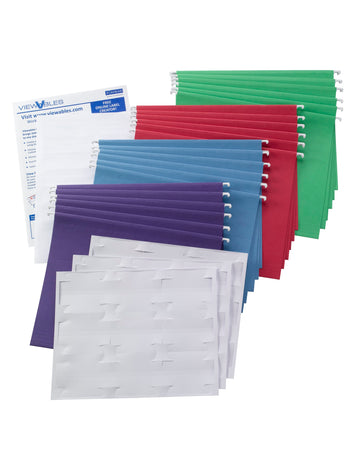This image depicts a neatly arranged set of colorful hanging file folders, typically used for organizing documents within a filing cabinet. The folders are grouped in sets of five, starting with green at the back, followed by red, light blue, and purple at the front. Each folder features white tabs that protrude from either side, designed for easy hanging and labeling. In the foreground are three white sheets, likely perforated labels meant for identifying the contents of the folders. To the left, two white pieces of paper are visible, with the back one partially covered and featuring small, unreadable blue text. The entire setup is arranged diagonally across a white backdrop, resembling a promotional image suitable for a catalog or a shopping website, such as Amazon, showcasing the vibrant color-coded organizational system.